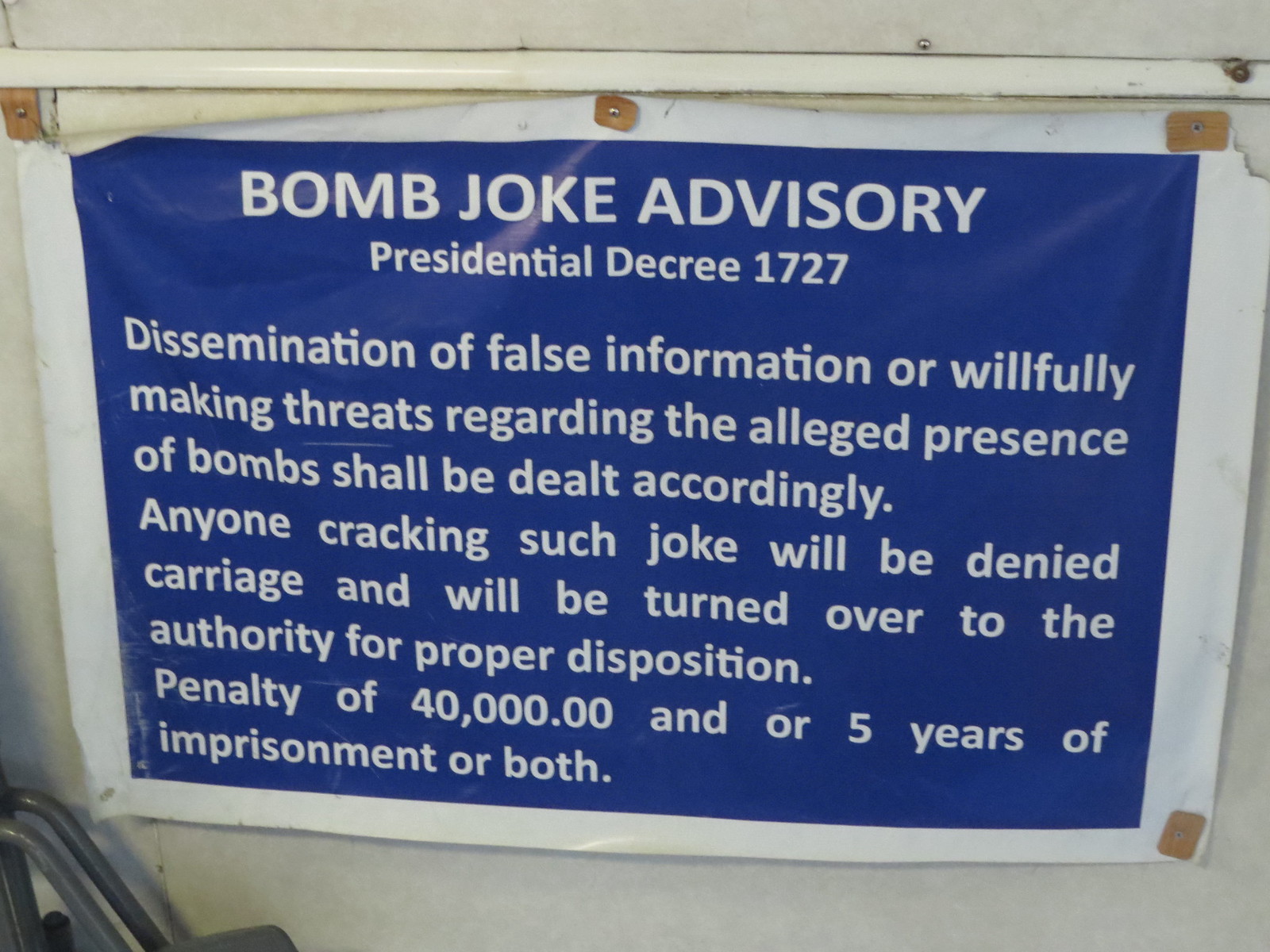The image depicts a beat-up informational sign nailed or screwed into a white wall. The sign, which appears to be made of plastic or a similar resilient material, has a white outline around its edges with a prominent blue background. The white text on the sign reads: "Bomb Joke Advisory, Presidential Decree 1727. Dissemination of false information or willfully making threats regarding the alleged presence of bombs shall be dealt accordingly. Anyone cracking such a joke will be denied carriage and will be turned over to the authority for proper disposition. Penalty of 40,000 and/or five years of imprisonment or both." The overall condition of the sign is quite worn, suggesting it has been in place for some time.